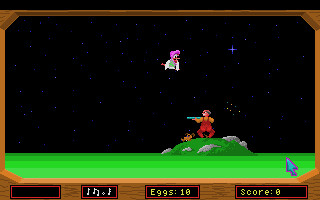This detailed caption for the image:

The image displays a screenshot from a video game. The primary screen is black, encased by a tan border. Below the main screen, there's a small wood-grain area featuring four distinct rectangles. These rectangles are black with red outlines. The rectangle on the far left is blank, the second rectangle contains music note symbols, the third rectangle displays "Eggs: 10," and the fourth rectangle reads "Score: 0."

In the game screen itself, the bottom quarter is dominated by a green landscape featuring a bright green hue with a slightly darker green mound adorned with flowers. Standing prominently on the mound is a hunter dressed in red overalls, wielding a gun. Higher up on the screen, there is a small blue cross, a plus sign, and an object resembling a duck.